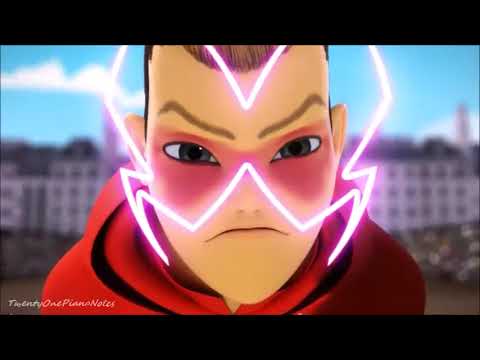This image showcases an animated character, possibly from a cartoon or video game, rendered with computer animation. The central character, a young white male with pale skin, is distinguished by his elongated, oval-shaped face and pointy chin. His slicked-back brown hair contrasts with his narrow, grayish-blue eyes, which are further accentuated by a red mask-like outline around them. His thin-lipped frown and prominent nostrils add to his stern expression, emphasized by his pinched-in eyebrows. The character wears a red hoodie with the hood down, and over his eyes, there is an illuminated, neon white goggle or faceplate. Positioned against a backdrop of a brightly blue sky with white clouds, the blurry, imposing shape of a large, white building can be discerned, suggesting a scene likely extracted from a video game or animated series.